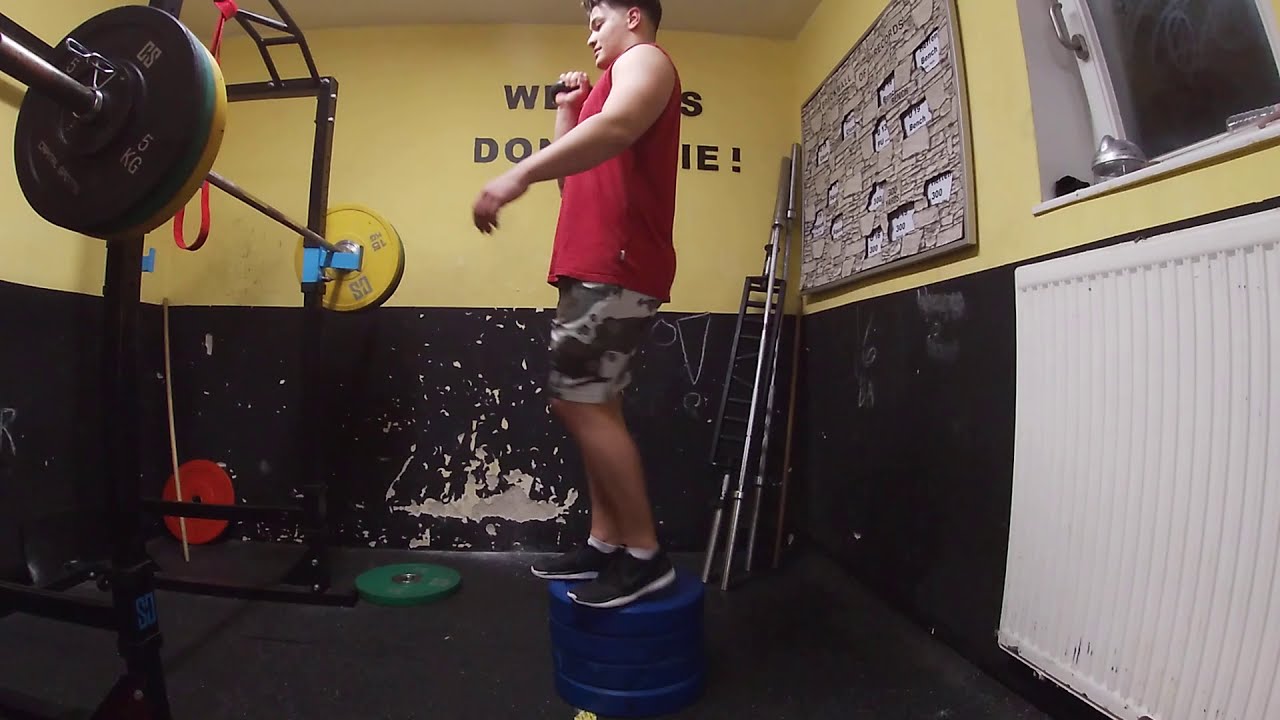The image captures a well-lit, detailed scene inside a small home gym. The walls of the gym are a vibrant yellow on the upper half and black on the lower half, showing signs of wear with chipped and gouged sections where the paint is missing. Prominent in the room is a young man with short dark hair and a lighter skin complexion, dressed in a red sleeveless shirt and dark green and beige camouflage-patterned shorts. He wears white socks with black shoes, standing precariously atop four stacked blue barbells, holding a small weight in his right hand, and balancing with his left arm slightly extended. He faces left, where a large metal stand supports a barbell loaded with four weights, two on each side. On the floor next to the stand, a green and a red weight lie individually. Behind him, partially obscured by his figure, is some black lettering on the yellow wall that remains illegible. To the right, a bulletin board and a small window with a radiator grill beneath it can be seen, adding functional elements to this home workout space. The clarity and color quality of the photograph are excellent, capturing every nuanced detail vividly.